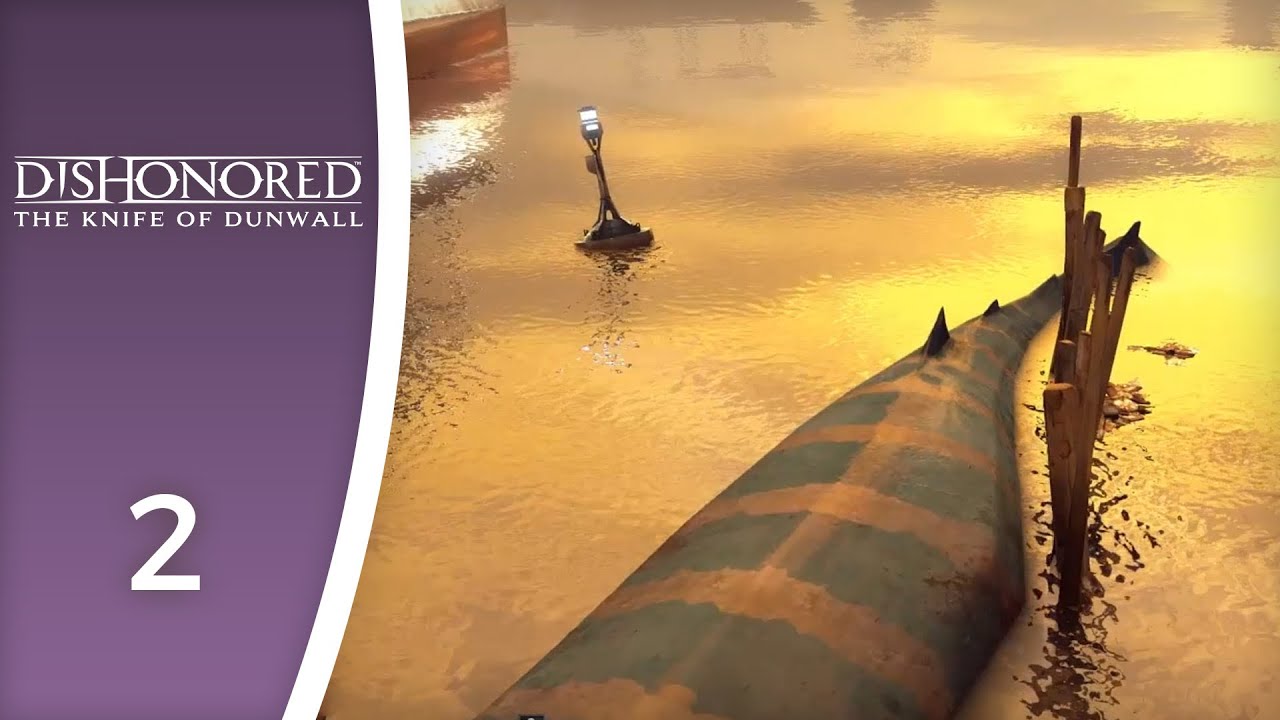This image, seemingly an advertisement or promotional poster, is divided into two distinct sections. The left section features a purple background with white text that reads "Dishonored, The Knife of Dunwall," followed by the number "2" at the bottom. A white border serves as a divider between the two sections. The right section portrays a sunset scene with hues of orange and yellow reflecting on a body of water. In the water, there is a lamppost or wood-like post and a large, mysterious creature or submarine-like object with an orange and black color scheme. The creature has distinctive details, which might resemble a dragon or another mythical animal, and there are hints of a fence or structure visible in the water, adding to the enigmatic ambiance of the scene.